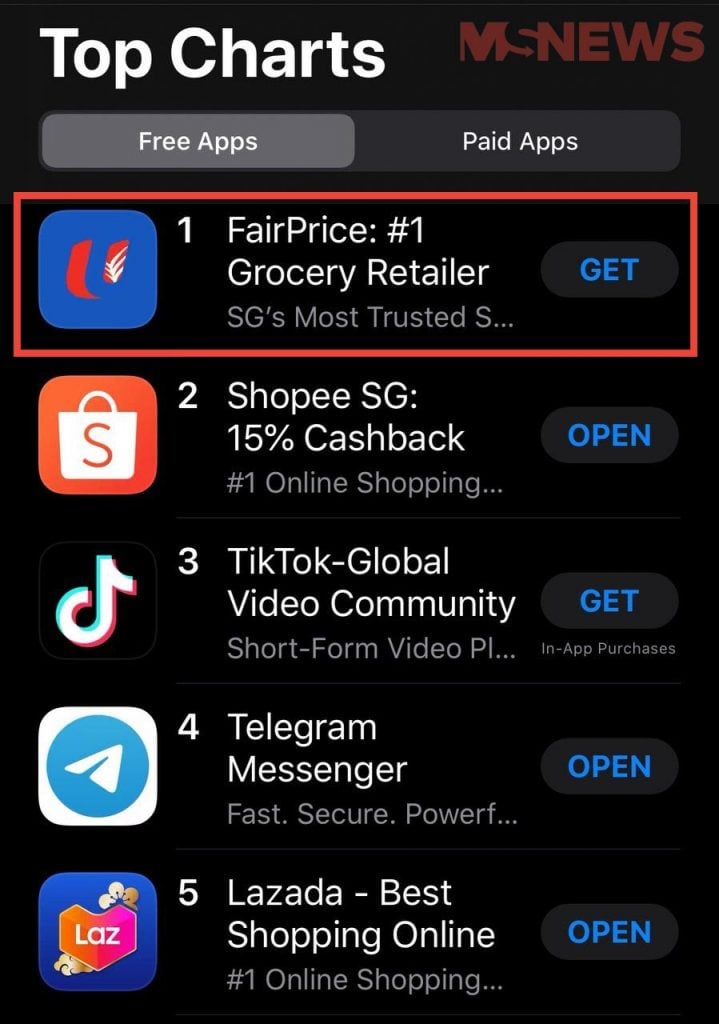This image is a screenshot displaying a section of an app store. The background is black. At the top right, there is the title "MS News" written in brown letters, except for the "S" which is black. In the top left corner, large white letters spell out "Top Charts." Below this, there are two tab options. The currently selected tab, "Free Apps," has white text on a grey background, while the adjacent tab, "Paid Apps," has white text on a dark grey background.

In the "Free Apps" section, the highlighted app is "FairPrice," outlined in a red rectangle. Its square icon is positioned on the left side, and it claims to be the "#1 grocery retailer." Additional text beneath the app name describes it as "SG's Most Trusted Shopping App." To the right, there is an oval button with blue capital letters that says "Get," indicating that users can download the app.

The list contains a total of five apps. The second app, "Shopee SG," is represented by a red square icon with rounded corners featuring a white shopping bag and the letter "S." It claims to offer "15% cash back" and has a button that says "Open," suggesting it's already installed on the device.

The third app is "TikTok," identified as the "Global Video Community." It has the recognizable TikTok icon on the left and a "Get" button, indicating it's available for download.

The fourth app, "Telegram Messenger," has an icon resembling a send arrow. The button for this app says "Open," indicating it's already installed on the device.

Finally, the fifth app is "Lazada - Best Online Shopping." Its icon is a blue square featuring a geometrical heart shape in orange and pink with the letters "L-A-Z" in the middle. There appears to be a background of cherry blossom flowers behind the heart. This app also has an "Open" button, indicating it's already installed on the device.